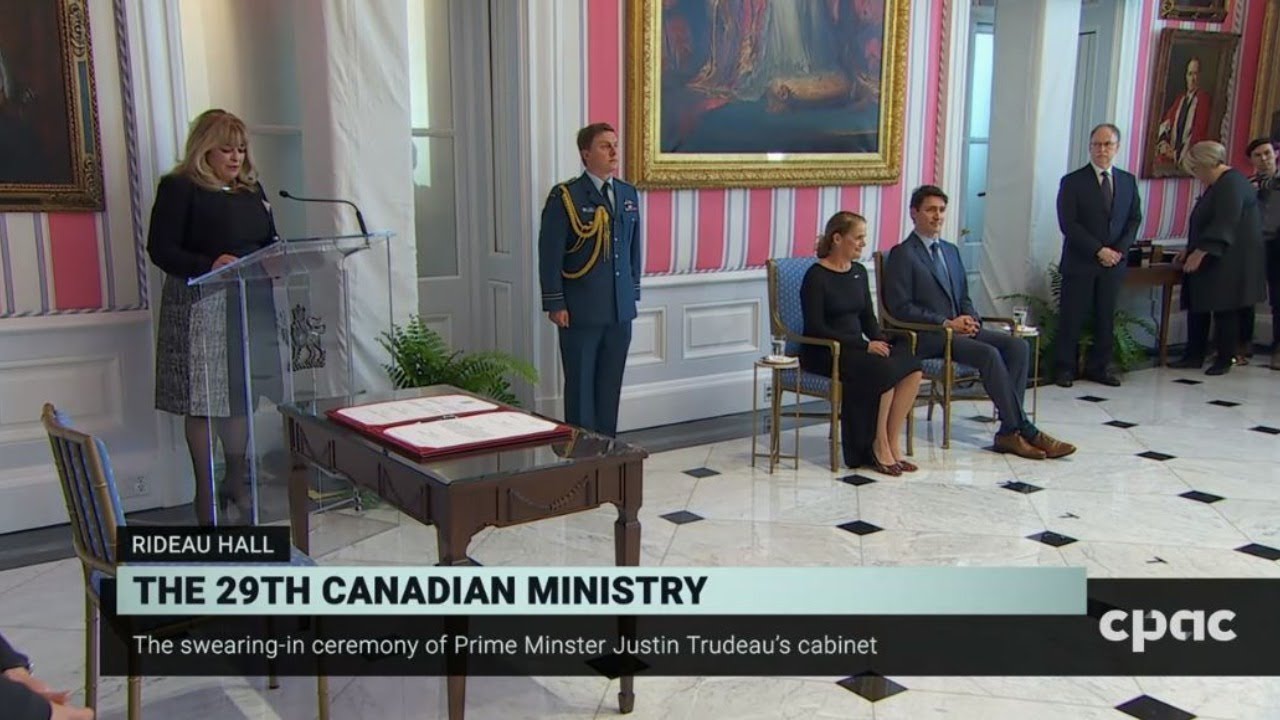The photograph captures the swearing-in ceremony of Prime Minister Justin Trudeau's cabinet, held at Rideau Hall, marking the formation of the 29th Canadian Ministry. The opulent stateroom features white walls adorned with pink and white stripes, large-sized oil paintings in gold frames, and a shiny white and black tile floor, conveying a palatial ambiance. Central to the scene are Justin Trudeau and his wife, both seated in ornate blue and gold chairs with folded hands. Trudeau, dressed in a dark blue suit with brown shoes and a blue tie, sits beside his wife, who is wearing a knee-length, long-sleeved dress with a scoop neck. To their right stands a dignitary in a navy blue uniform with gold braid, maintaining a posture of attention. At a glass podium with a microphone, a woman with blonde shoulder-length hair, dressed in a dark top and gray print skirt, addresses the assembly. In front of her stands an antique brown desk with two large pieces of paper mounted on red material. This formal moment is underscored by the text label at the bottom of the image, which reads, "Rideau Hall, the 29th Canadian Ministry, the swearing-in ceremony of Prime Minister Justin Trudeau's cabinet." The scene is framed within the context of a news broadcast, as indicated by the CPAC logo in the lower right corner.